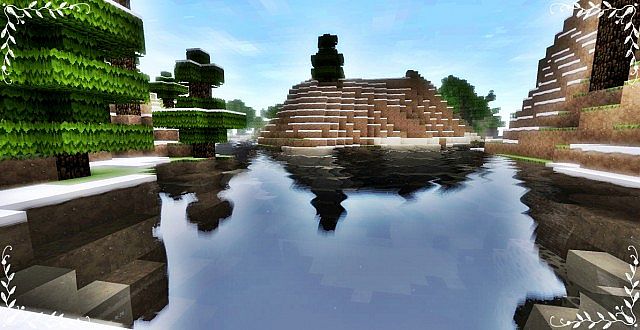This detailed image is a computer-generated screenshot from the game Minecraft. It showcases a three-dimensional scene centered around a small, pixelated lake. Surrounding the lake are stepped, blocky monuments that rise towards the sky, with some covered in snow and others topped with green tiles. To the top left corner of the image, there are squarish, green trees with brown trunks that exhibit an artificial, unrefined appearance typical of Minecraft's blocky aesthetic. The sky is light blue with scattered clouds. The water surface appears slightly pixelated and reflects the surrounding landscape, casting shadows of the trees and monuments. Additionally, white ivy decorates the corners of the image, and the underwater ground mirrors the color and texture of the land above.